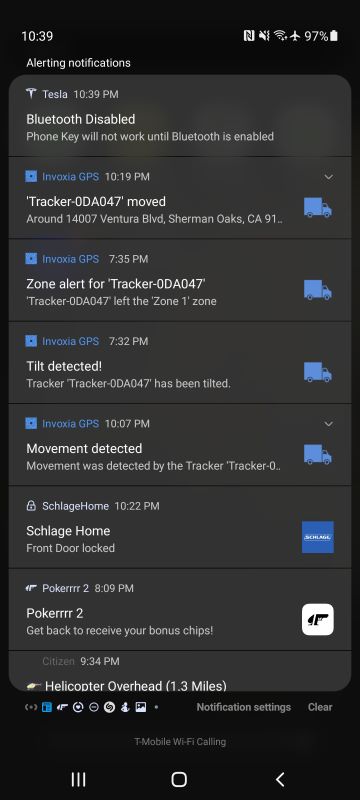This is a detailed screenshot captured from a mobile phone with a black background. At the top, in white font, the time reads 10:39 PM. A series of status icons appear below the time, indicating that the phone's sound is off, Wi-Fi signal is at full strength, Airplane mode is activated, and the battery is at 97% charge.

Below this status bar, a heading reads "Alerting Notifications," followed by eight notifications displayed in little gray rectangles.

The first notification, timestamped at 10:39 PM from Tesla, indicates: "Bluetooth disabled. Phone key will not work until Bluetooth is enabled."

The second notification, from Anoxia GPS at 10:19 PM, states: "tracker-odaq47 moved around 1407 Ventura Boulevard, Sherman Oaks, California, 9-1."

The third notification, also from Anoxia GPS at 7:35 PM, reads: "Zone alert for tracker-odaq47. Tracker-odaq47 left the zone 1 zone."

The fourth notification from Anoxia GPS at 7:32 PM simply declares: "Tilt detected."

This descriptive caption clearly outlines the detailed content present in the screenshot, capturing all the essential elements and notifications displayed on the device.